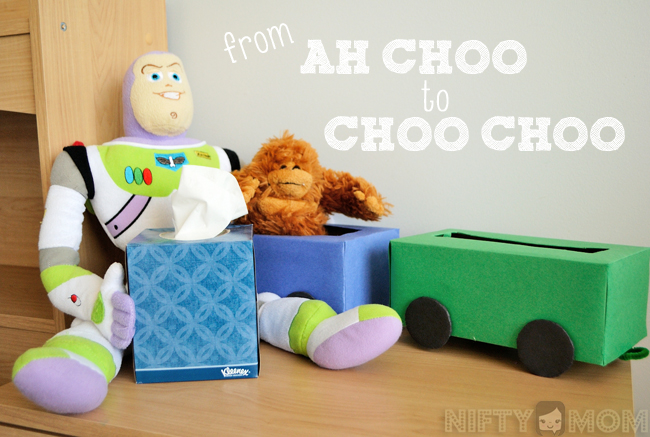The image depicts a whimsical advertisement for a toy-themed tissue box setup against a gray wall with the prominent white lettering that reads "From Achoo to Choo Choo." At the center of the scene is a Buzz Lightyear doll seated on a light brown wooden desk. Buzz is holding a blue Kleenex tissue box with a tissue extending from it. To his side, there is a playful train crafted from tissue boxes; the blue car, which has a slit for tissues, contains a stuffed gorilla, while the green car behind it features black wheels. Buzz leans casually against the blue train car, seemingly wrapping an arm around the gorilla, adding a friendly, interactive touch to the display. The image also bears the logo "Nifty Mom" with an illustration of a mother figure situated between the words "Nifty" and "Mom."